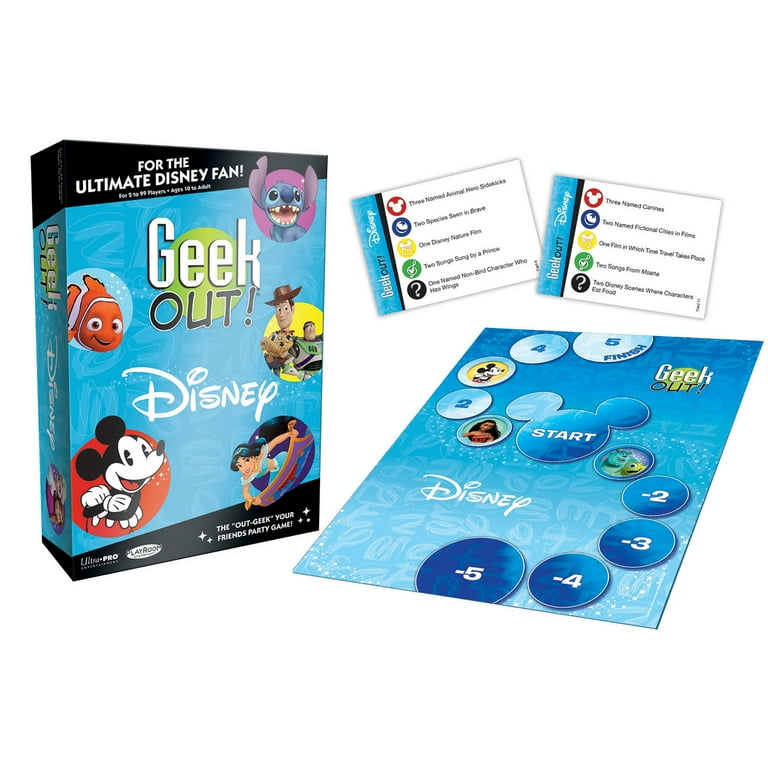The image displays a Disney-affiliated card game titled "Geek Out" designed for the ultimate Disney fan. The game packaging features a prominent blue and black color scheme with a green logo where "Geek" is written in white and "Out" in black. The top of the box declares the game is "For the Ultimate Disney Fan" in white text on a black background. The box showcases a variety of beloved Disney characters including Nemo from Finding Nemo, Stitch from Lilo & Stitch, Woody and Buzz Lightyear from Toy Story, Mickey Mouse, and Jasmine from Aladdin on her flying carpet. The lower section of the box describes it as "The Out-Geek Your Friends Party Game." To the right side, there are trivia categories like “Three Named Animal Hero Sidekicks,” “Two Species Seen in Brave,” and “One Disney Nature Film” displayed on colorful cards. The game also includes a board mat with positive and negative numbered circles leading from "Start," featuring Disney character illustrations where players presumably move their pieces as they answer trivia questions.